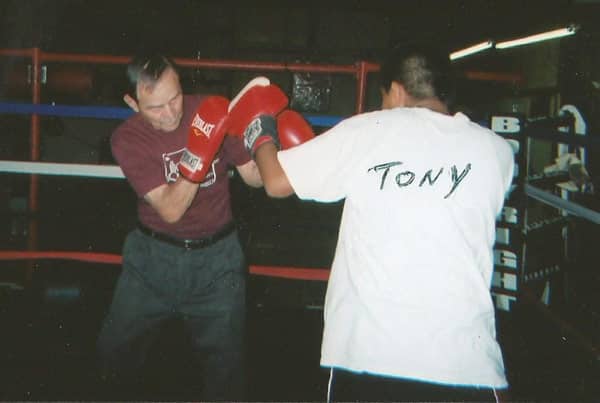This appears to be a vintage, low-quality photo, likely taken with a Polaroid camera, capturing a boxing training session in what seems to be a dimly lit boxing gym from the 1970s or 1980s. The photograph shows two men engaged in boxing, presumably a boxer and his trainer. The older man on the left, sporting a maroon shirt, dark grey pants with a black belt, and boxing gloves, has his hands up in a fighting stance. He has a stern and focused expression, indicative of his role as the trainer. The boxer, facing away from the camera, wears a white t-shirt with the name Tony handwritten on the back, as well as black shorts and red boxing gloves. Behind them, two boxing rings are visible, one with red, blue, and white ropes and the other with black, grey, and white ropes, adding to the gym's authentic atmosphere. The ambient light captures faint color details, enhancing the nostalgic feel of the scene.